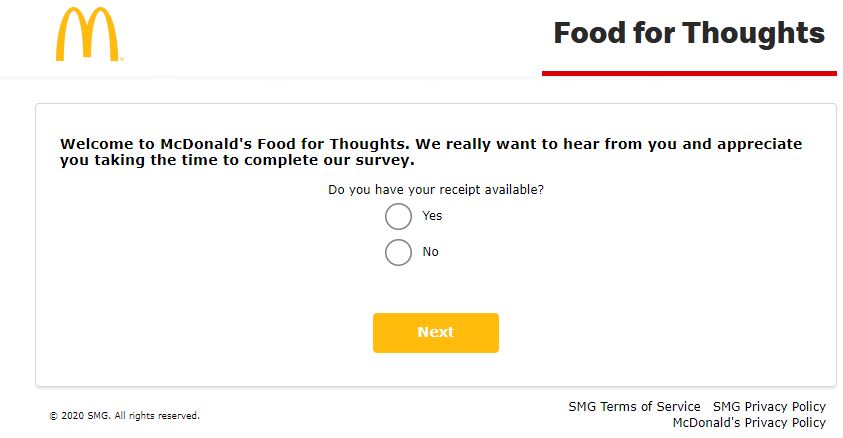This image captures a section of a McDonald’s customer survey website, identifiable by the prominent McDonald's logo ("M") on the left side. On the right, the phrase "Food for Thoughts" is distinctly underlined in red. The visible portion of the webpage appears to be an introductory segment of a customer survey, which reads: "Welcome to McDonald's Food for Thoughts. We really want to hear from you and appreciate you taking the time to complete our survey." Below this message, the survey prompts the user with the question, "Do you have your receipt available?" with options for "Yes" or "No." Beneath this question is a noticeable gold button labeled "Next." The image suggests that upon completing the survey, customers might receive a code on their receipt, which can be redeemed for a discount or a free item—a common practice noted here. The text also indicates that this particular survey page is from the year 2020.